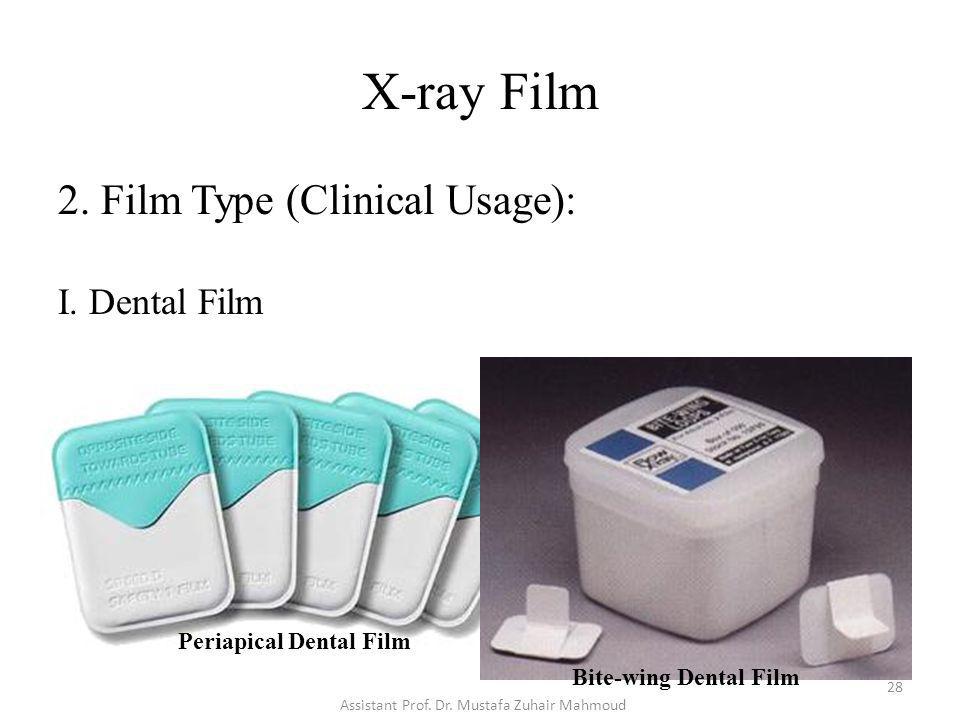The image appears to be an educational slide or possibly an advertisement from a medical website or textbook. The slide is titled "X-ray Film," and it features detailed information and visuals on different types of dental X-ray films. Below the title, the text reads: "2. Film Type (Clinical Usage):" followed by "I. Dental Film." 

On the left side, there is a depiction of "Periapical Dental Film," illustrated with an image of the product, which appears as a thin sheet with the top half colored light blue and the bottom half white. On the right side of the slide, another type labeled "Bite-Wing Dental Film" is shown. This product is displayed as a small rectangular piece of plastic designed to be bitten into, with a clear container holding additional pieces. The background colors of the slide include turquoise, blue, black, white, and gray tones. The image is in an upright position, with some items stacked and fanned out, suggesting an organized arrangement typical of educational resources or professional advertisements. Additionally, the name "Assistant Professor Dr. Mustafa Zuhair Mohamed" is mentioned, indicating an authoritative source or contributor to the slide's content.